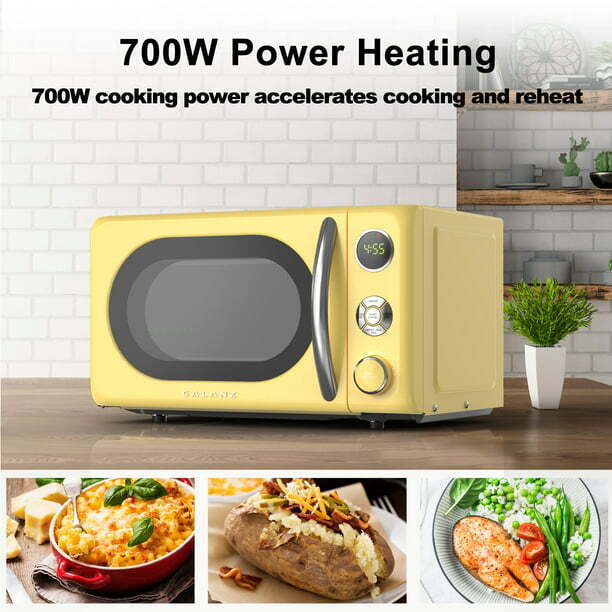The advertisement showcases a retro-styled, yellow "Galant" microwave oven, with an oval-shaped viewing window and a sleek silver handle, exuding a distinct 1950s vibe reminiscent of the Fallout video game universe. Positioned on a wooden table against a white brick wall, the microwave has a prominent circular LED display indicating the time in green, flanked by buttons and a control knob beneath. At the top, the ad highlights its "700W power heating" and "700W cooking power accelerates cooking and reheat" capabilities in black text. The bottom portion of the ad features three images of dishes prepared using the microwave: a red tray with mac and cheese, baked potatoes with creamy toppings, and a plate of chicken with an assortment of vegetables, including peas and tomatoes.